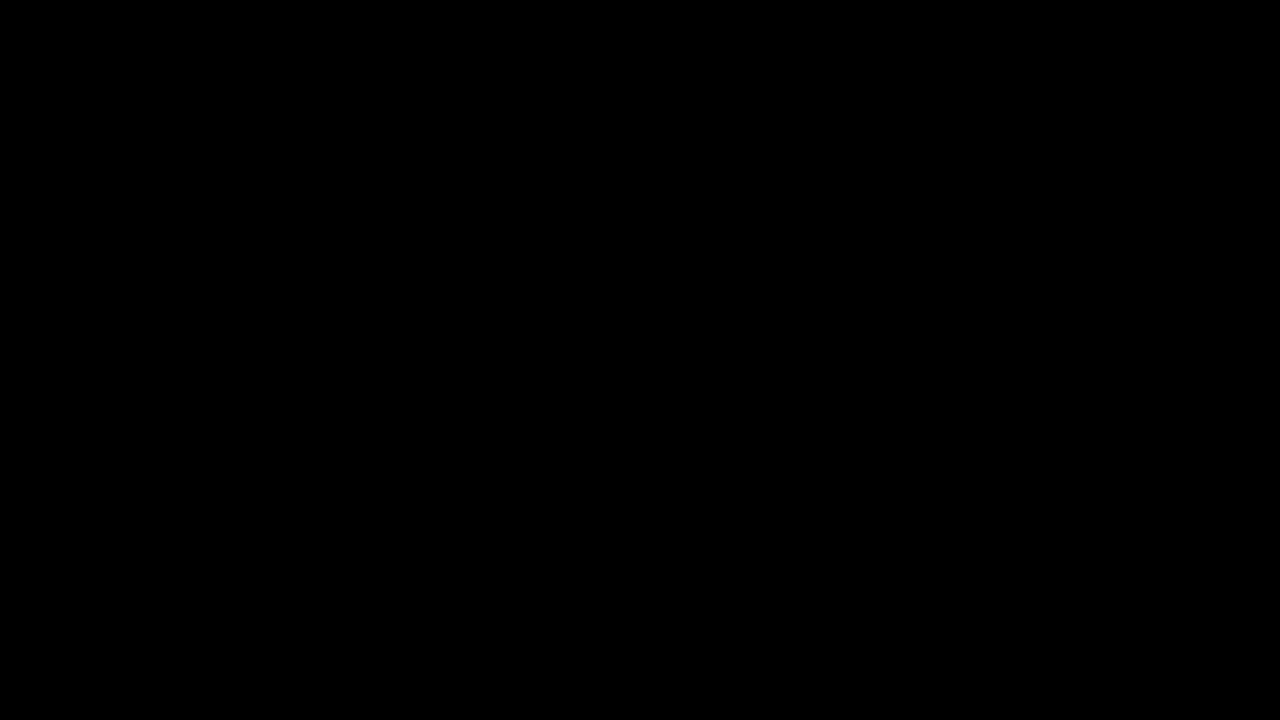The image is an extremely simplistic, solid black rectangle with no visible details or elements whatsoever. It's in landscape orientation, with perfect 90-degree angles forming its boundaries. The absence of gradation, light, or any distinguishable features makes it a flat, jet-black surface. There's no hint of text, graphics, borders, or icons, making it appear as if the image might not have loaded correctly. The overall effect is an expanse of pure black, devoid of any focal point or area of interest, potentially resembling a darkened room rather than the night sky, given the absence of stars or other distinguishing features.